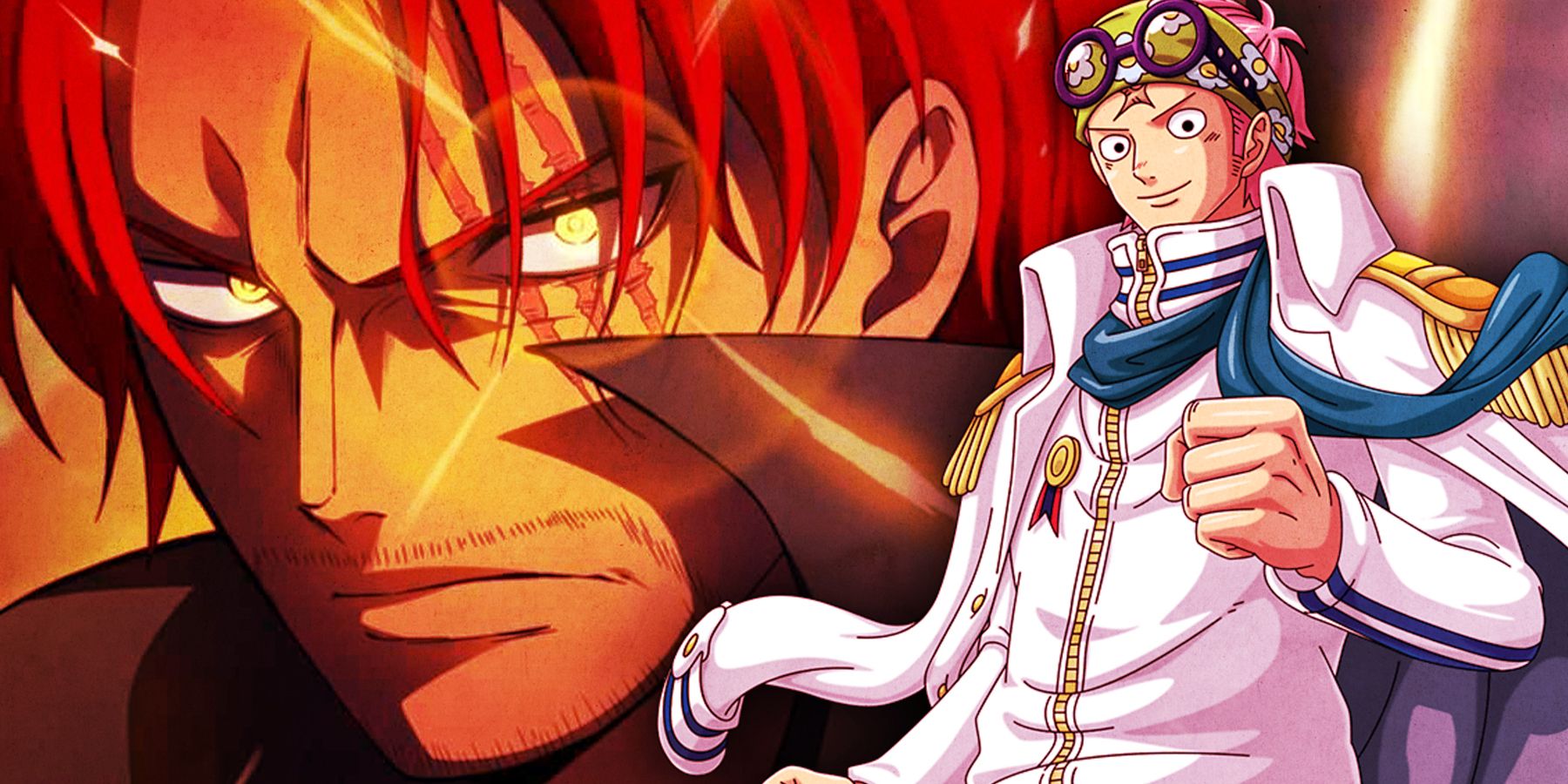In this animated image from the series One Piece, a dramatic scene unfolds featuring two notable characters. Dominating the background is Shanks, who strikes an imposing figure with his red hair draped over his forehead, a thin mustache, and beard. His face, accentuated by three distinct scars over his left eye, is captured in a close-up, shrouded in hues of orange and red. His eyes, piercing and menacing, have a glowing yellow hue, adding to his intense demeanor. He is adorned in a high-collared garment, the details of which blur into the background due to the close zoom.

To his right stands another character, identifiable by his iconic yellow bandana with white flowers. He sports a pair of purple goggles perched above his eyes and a cheerful smile. His attire is striking: a white naval uniform featuring a large collar, gold shoulder pads with tassels, a blue scarf, and a ribbon on his chest. His left hand is lifted in a fist, exuding confidence. His pink hair adds a vibrant touch to his appearance, making him easily recognizable to long-time fans of the series.